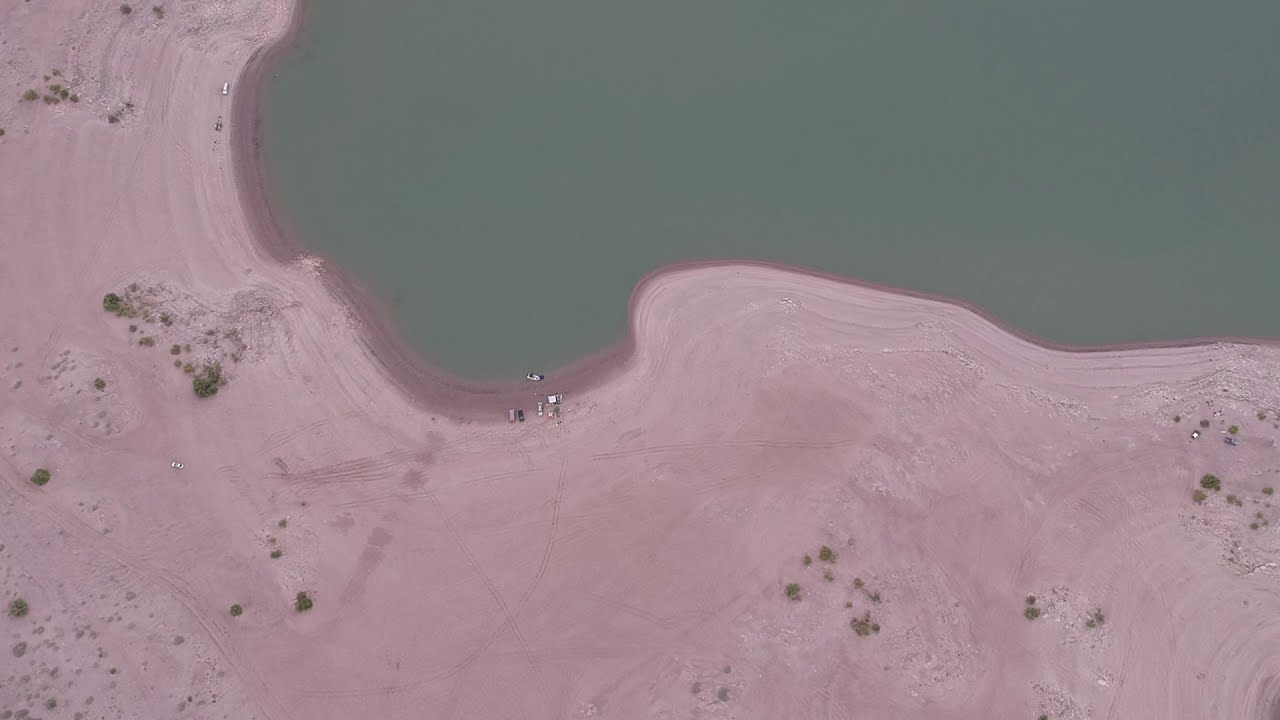This is a high-angle, aerial view of a desolate beach scene captured in a horizontally aligned rectangular photograph. The landscape is split between a sandy area and a body of water. The expansive sandy terrain occupies the bottom left portion to the middle right of the image and appears light pinkish or purplish with scattered green patches, which seem to be sparse vegetation. The sand transitions to a darker brownish-gray hue along the edges where it meets the water.

At the upper part of the image, the water body stretches from the upper right, curves down and across the middle, then arcs upward towards the upper left. The water appears flat and changes in color from greenish-gray to a more consistent gray tone. Near the center, slightly to the left, a group of vehicles is visible, akin to tiny matchbox cars, indicating how high up the photograph was taken. This detail adds a sense of scale to the otherwise vast and sparse environment. 

No textual elements are present in the image.